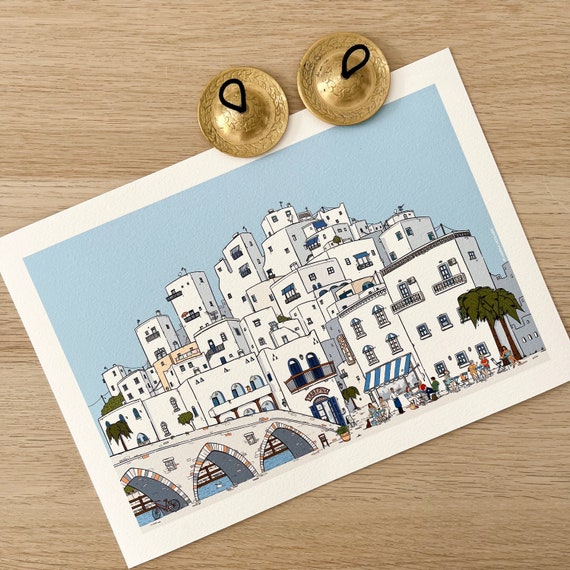This image depicts a detailed scene of a picturesque and intricate European, possibly Mediterranean or Italian, city set against a light-colored, brownish or oak table top. Sitting atop the picture on the table are two gold-colored circular objects with black loops, possibly bells, indicating a decorative touch. The picture itself is potentially a print, watercolor, or postcard showcasing the cityscape with white buildings, some adorned with blue and white awnings. These structures vary in shape but are predominantly square with slight variations in features and are densely packed together.

A prominent bridge with three arches stretches across water, adding depth to the composition. Underneath one of the arches, a red bicycle is propped up, providing a pop of color. To the left of the bridge, a solitary tree can be seen, and another tree is present on the right-hand side, contributing to the green elements in the scene. Additionally, there is an open-air restaurant depicted in the lower right corner with several people seated at tables, possibly enjoying a meal, and a waiter serving them. This scene captures the idyllic charm and bustling life of a quaint coastal town.